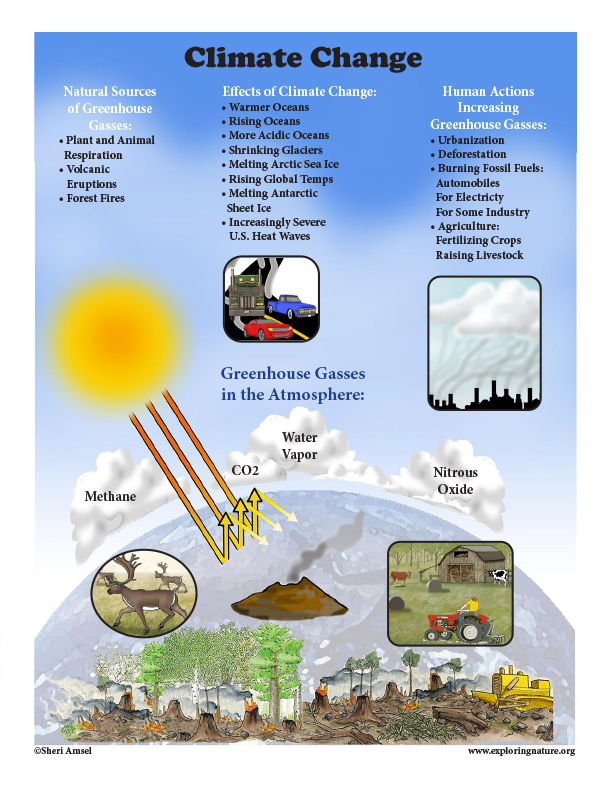This is an informational poster on climate change, featuring a detailed diagram with a darker blue background fading to lighter blue, and a central gray sphere representing the Earth. At the top, "Climate Change" is written in bold black letters. The diagram is divided into three main sections, each explaining different aspects of climate change.

On the upper left, the white text highlights "Natural Sources of Greenhouse Gases." Below, in black bullet points, it lists:
- Plant and animal respiration
- Volcanic eruptions
- Forest fires

In the center, under white font reading "Effects of Climate Change," black bullet points enumerate:
- Warmer oceans
- Rising oceans
- More acidic oceans
- Shrinking glaciers
- Melting Arctic sea ice
- Rising global temperatures
- Melting Antarctic sheet ice
- Increasingly severe US heat waves

Below this section, an image depicts a red car, a blue pickup truck, and a green semi-truck skidding down a mountain road.

On the upper right, white text introduces "Human Actions Increasing Greenhouse Gases." In black bullet points, it lists:
- Urbanization
- Deforestation
- Burning fossil fuels
- Automobiles
- Electricity for some industries
- Agriculture
- Fertilizing crops
- Raising livestock

Beneath this section, a silhouette of smokestacks emits gray smoke into large clouds. 

Below the central image, blue text says "Greenhouse Gases in the Atmosphere." An illustrated sun to the left sends arrows towards Earth, which then bounce off and are reflected back by clouds labeled CO2, Methane, Water Vapor, and Nitrous Oxide. 

A circular inset shows two male deer walking to the left. Next to it, an illustration depicts a volcano emitting smoke. Below this are images of deforestation with a red tractor and a farm scene with a farmer, cows, and a forest transitioning from green to brown.

At the bottom left corner, "Copyright Sherry Armcell" is noted, while the bottom right corner cites www.exploringnature.org.